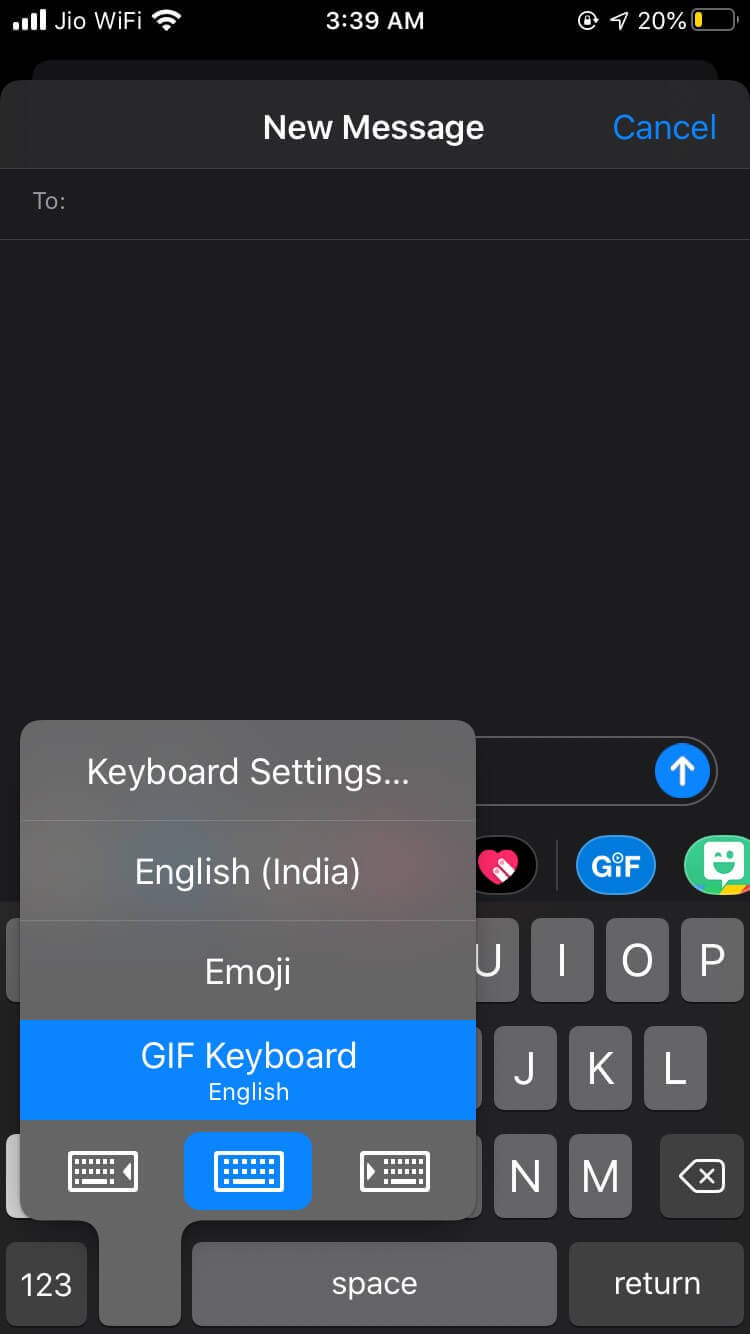Screenshot of a smartphone displaying a variety of on-screen elements. The status bar at the top shows a strong Wi-Fi connection labeled "J-Lo Wi-Fi" with all four bars filled, indicating excellent signal strength. It is 3:39 AM and the battery is at 20%, highlighted in yellow. A white notification reads "New Message," with a blue "Cancel" option adjacent to it. Below this, the number "2" is visible, suggesting possibly a message count or selection. The background of the display is black.

Towards the bottom of the screen, there is a section labeled "Keyboard Settings" listing options such as "English (India)," "Emoji," "Gift Keyboard," with "English" highlighted in blue.

Part of the keyboard is visible, showing letters from "U" to the right, along with various other keys such as a heart symbol, an oval-shaped gift button, and a talk button. The bottom row includes numbers "1, 2, 3," a tab key for keyboard settings, a space bar, and a return key. The image overall provides a detailed view of the phone's current connection, battery level, message notification, and keyboard customization options.